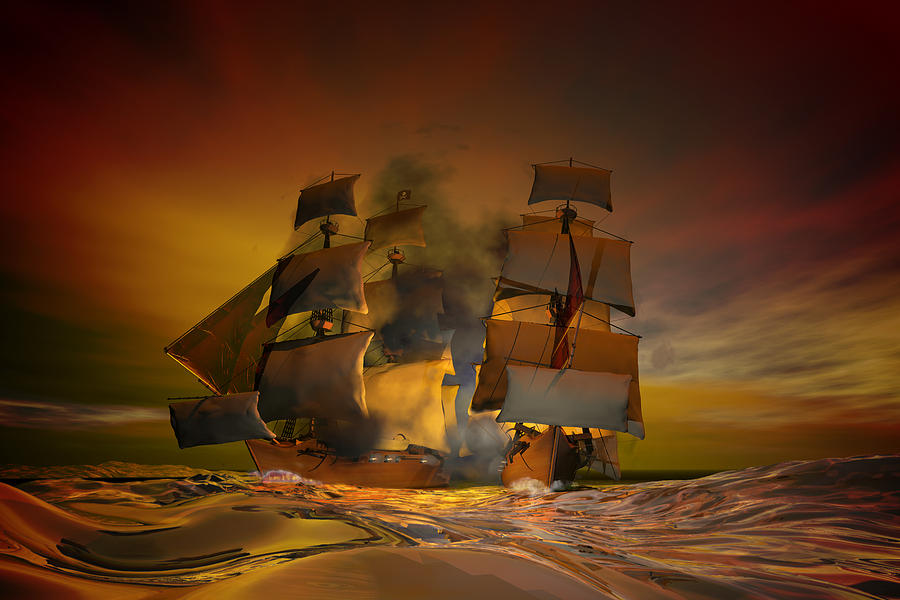The image is a computer-generated artwork in a horizontal rectangular frame, depicting the catastrophic aftermath of a violent oceanic conflict. An old pirate ship, rendered in an array of brown, dark red, and dark yellow hues, is dramatically ripped in half and on the verge of sinking into the turbulent sea. Surrounding the ship, the water echoes the scene's somber palette with dark red and brown tones. Another wooden vessel, similarly designed, floats nearby, compounding the chaos. The vessels' immense sails, now tattered, are dark gray, while billows of thick, dark gray smoke rise hauntingly from the centers of both ships, suggesting recent explosive damage or fire. The sky is painted in a gradient of bronze, orange, and dark red, transitioning into dark gray, evoking the time of day when twilight takes over and amplifies the scene's apocalyptic mood. The ocean waves, detailed and reflective, add to the sense of turmoil and disaster, making it clear that this is a devastating and highly animated pirate battle frozen in time.